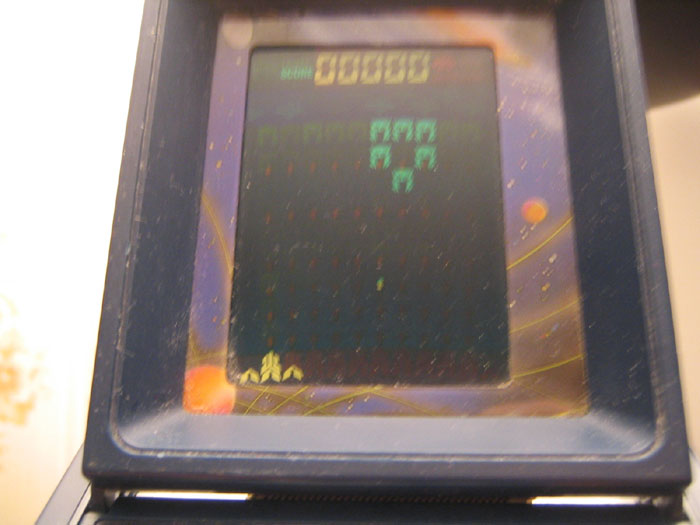The image shows a close-up of an old-style video game screen, likely a handheld gaming device or a small arcade console. The screen, which is somewhat dusty, features a row of six green enemies at the top arranged in two rows of three, with one enemy appearing to dive into the lower row. The score displayed at the top reads "000000." At the bottom left of the screen, there is a gun turret comprised of three shapes, presumably for shooting at the enemies. A decorative blue space-themed border surrounds the screen, adorned with orange planets, stars, and streaks, adding to the galactic theme. The background is blurry and possibly a white wall, but it is difficult to discern distinct details.